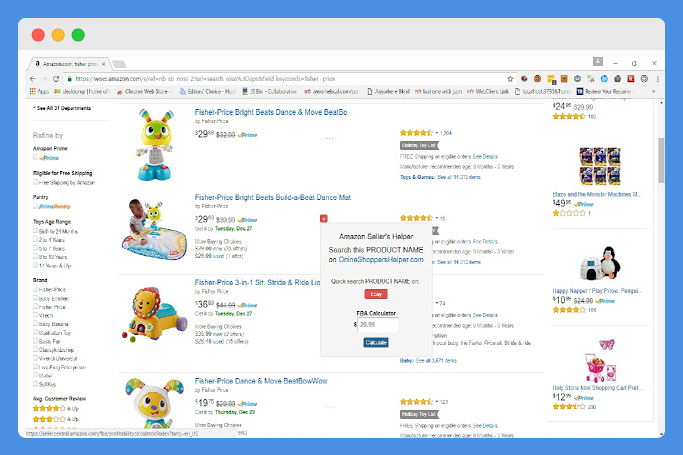The image is a screenshot of an Amazon storefront taken on a MacBook using a Google Chrome browser. The background of the screenshot is a light blue color, while the window of the Google Chrome browser has a predominantly white background. The screenshot quality is quite blurry, making most of the text difficult to read. However, a pop-up window is visible on the screen, reading "Amazon Sellers Helper. Search this product name on online shoppershelper.com." Additionally, the pop-up includes the options for a quick search product name and a small, unreadable red bar, followed by tabs labeled "FBA Calculator" and "Calculate" in blue.

In the background, several products are visible, predominantly children’s toys. The first product featured is the "Fisher-Price Bright Beats Dance & Move BeatBowWow," showcasing a colorful toy with blue, yellow, and green elements. The second item is the "Fisher-Price Bright Beats Build-a-Beat Dance Mat," depicted with a small child sitting on the mat and the BeatBowWow toy beside them. The third product listed is the "Fisher-Price 3-in-1 Sit, Stride & Ride Lion," which is a small rideable toy in yellow, blue, and red colors. The fourth product shown is the "Fisher-Price Dance & Move BeatBowWow," a toy distinguished by its yellow, white, and blue colors.

The screenshot also features a bookmark bar crowded with numerous, difficult-to-read bookmarks. Additional products are scattered around the screen, with a filter panel on the left-hand side. This panel allows users to refine their search based on brand, average customer review, and other criteria.